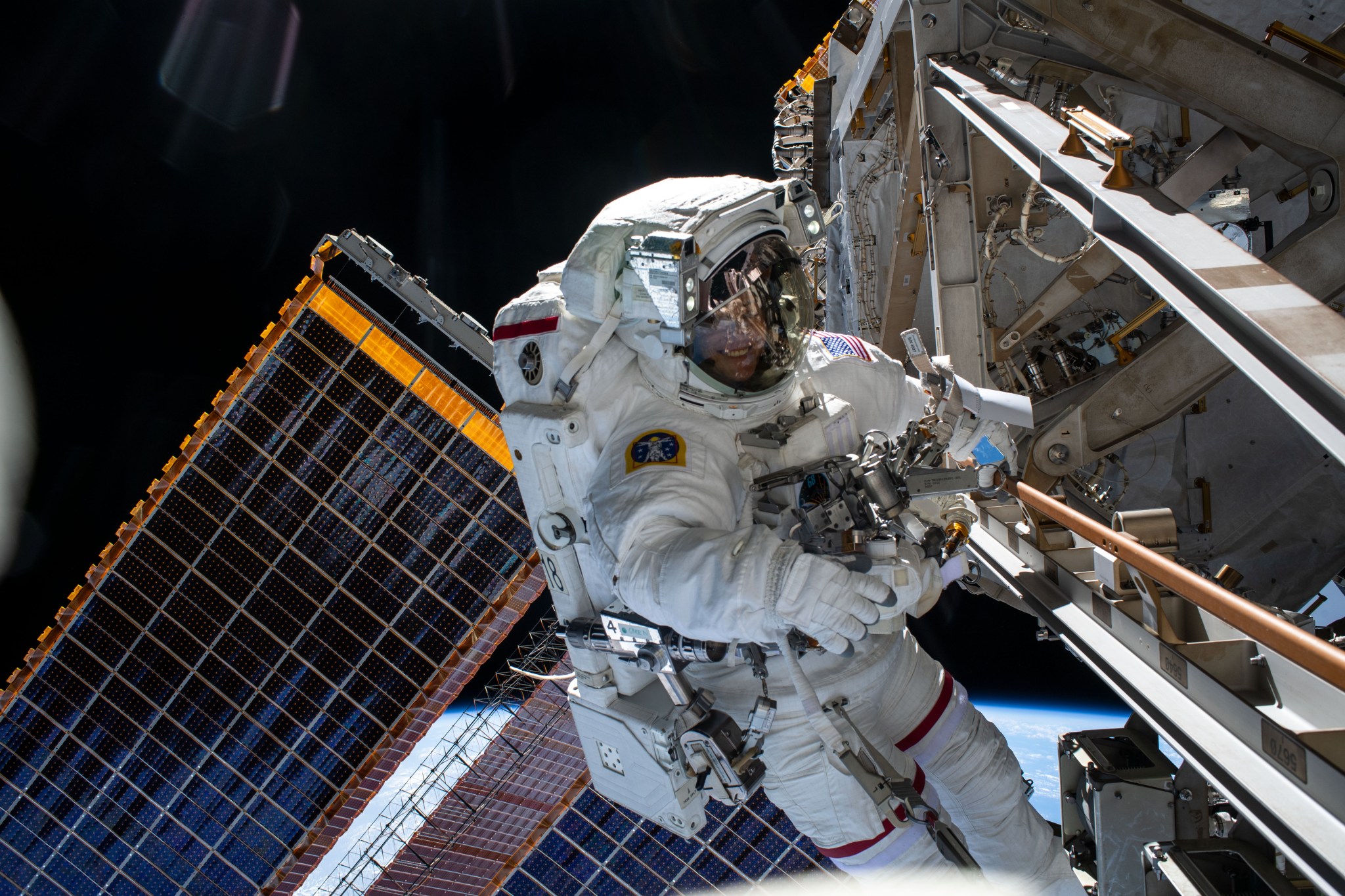In this stunning horizontal rectangular photograph taken outside the International Space Station, an astronaut in a full white space suit is performing an EVA (Extravehicular Activity) to conduct repairs on a solar panel. The astronaut's white suit, complete with a large backpack housing life support systems, and a helmet with a clear plexiglass visor, protects them from the harsh environment of space. Through the visor, a faint smile is visible, partially reflecting the surrounding machinery. The background showcases the vast blackness of space, with a faint glimpse of Earth at the bottom of the scene. Behind the astronaut, multiple large solar panels are visible, some being meticulously inspected and manipulated, suggesting intricate repair work on one of them. Ambient sunlight softly illuminates the scene, casting reflective glints off the astronaut’s visor and suit, providing a beautiful contrast to the otherwise dark surroundings.